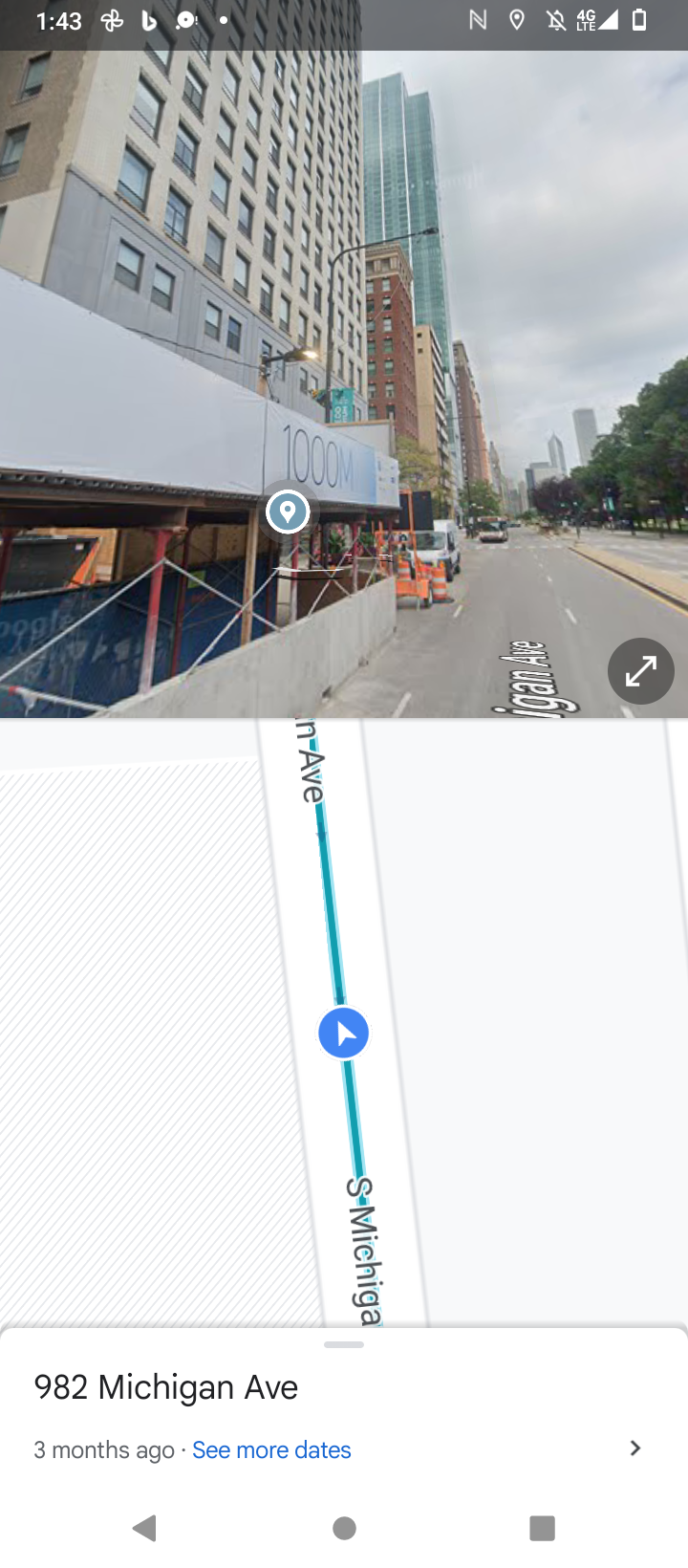This image is a detailed phone screenshot taken at 1:43, evident by the clock on the top of the screen alongside standard phone icons like GPS, 4G LTE, signal bars, and battery status. The upper portion of the screenshot showcases the Google Maps interface in Street View mode, displaying a real-time view of a cityscape. Lining the left side of the road are a series of tall buildings, presumably skyscrapers, with a few trees visible to the right. The cloudy, white sky dominates the background, casting a muted light over the scene. A prominent pin marks a building on South Michigan Avenue with the address 982 Michigan Avenue. Below the image, a navigation bar shows a long white rectangle with a teal strip and a blue circle containing a triangle, labeled “South Michigan.” Further details indicate the data was captured three months ago, with an option to "see more dates" in blue. The bottom part of the screenshot reveals map directions suggesting a straightforward route along South Michigan Road, with various directional icons like an arrow, circle, and square for additional functionality.